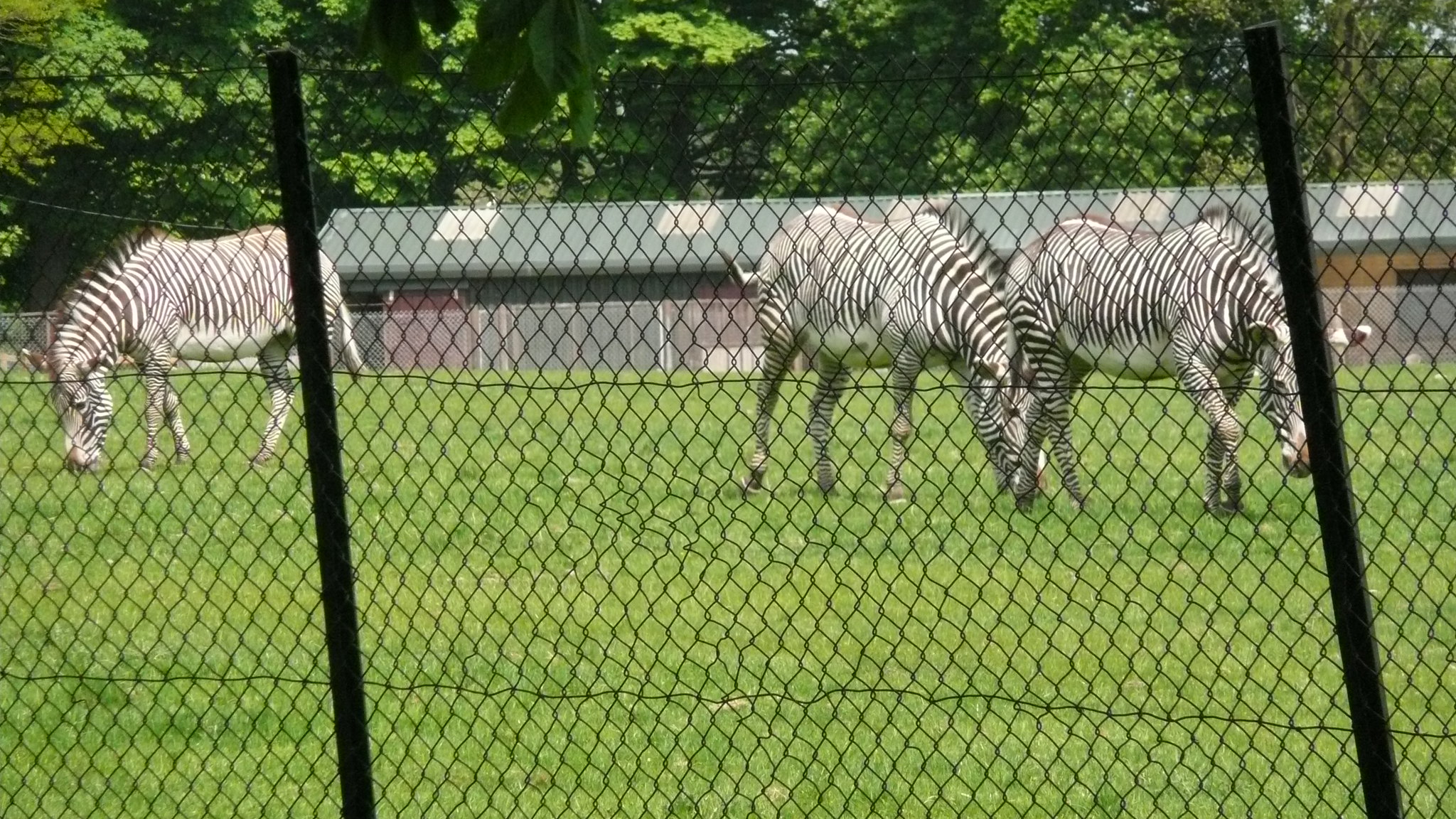The image captures three black and white adult zebras grazing in a lush green field, taken through a black chain link fence with visible posts. Two zebras are positioned to the right, one slightly behind the other, while the third stands to the left with its head near the left corner of the frame. The zebras are surrounded by a field enclosed by a black wire mesh fence. In the background, a long, low barn with a green roof features evenly spaced skylights or clear roofing material, and possibly pink doors. Beyond the barn, a forest of mature, green deciduous trees forms a scenic backdrop. The zebra on the far right grazes with its head raised slightly, contrasting with the others who are all engrossed in feeding. The scene evokes a serene moment of the animals in a controlled, possibly sanctuary-like environment.